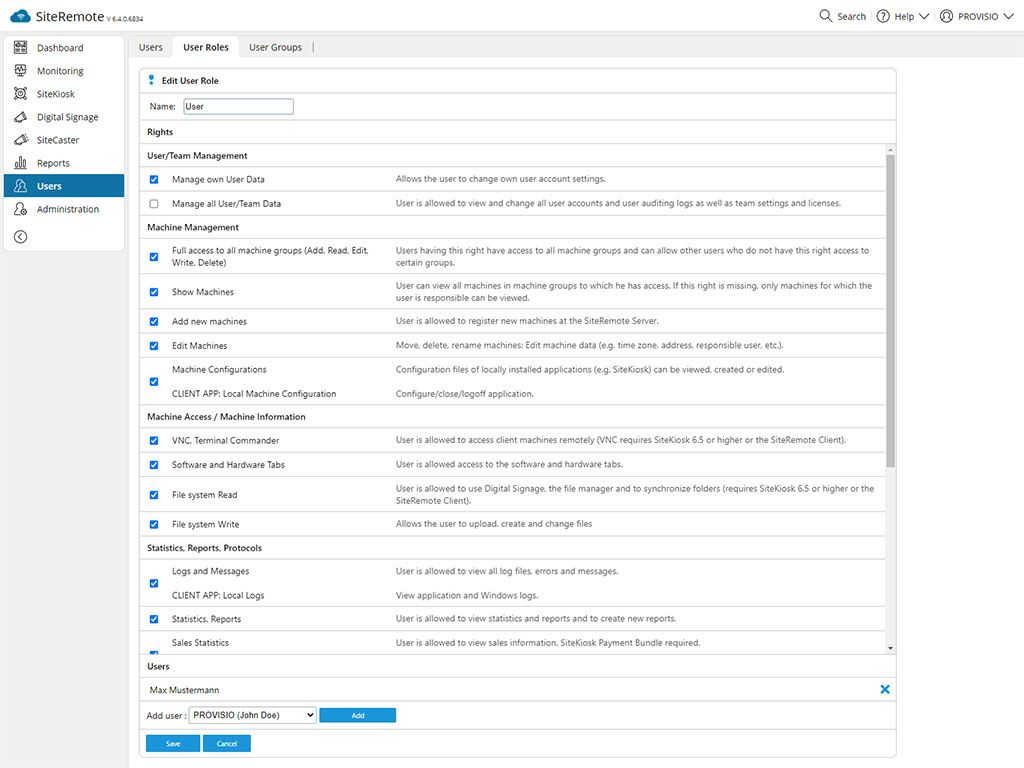**Descriptive Caption:**

The image features a detailed interface of a software management dashboard labeled "Site Remote." The top left corner displays the "Site Remote" title, while the top right features options for "Search," "Help," and "Provisio." The left side hosts a vertical menu with multiple sections: "Dashboard," "Monitoring," "Site Kiosk," "Digital Signage," "Site Caster," "Reports," "Users," and a highlighted "Administration."

To the right of this vertical menu is a horizontal menu bar with options "Users," "User Roles" (which is highlighted), and "User Groups." Below this menu bar is the section titled "Edit User Role," with sub-sections including "Name: User" and "Rights: User Team Management," followed by specific permissions detailed as follows:

1. **Manage Own User Data** (Checked): Allows the user to change their own account settings.
2. **Manage All User/Team Data**: Gives the user the ability to view and change all user accounts, user auditing logs, and team settings and licenses.
3. **Machine Management**:
   - **Full access to all machine groups** (Checked): Users can add, read, edit, write, and delete machine groups, and allow other users specific access.
   - **Show Machines** (Checked): Allows the user to view all accessible machines and groups.
   - **Add New Machines** (Checked): Permits registration of new machines to the server.
   - **Edit Machines** (Checked): Enables moving, deleting, renaming machines, and editing machine data like time zone, address, and responsible user.
   - **Machine Configurations** (Checked): Users can view, create, or edit configuration files for locally installed applications.
   - **Configure/Close/Log off Application**: [Specific permissions not detailed].
   - **Machine Access/Machine Information**:
     - **VNC Terminal Commander** (Checked): Grants remote access to client machines (requires Site Kiosk 6.5 or higher or the Site Remote client).
     - **Software and Hardware Tabs** (Checked): Allows access to software and hardware tabs.
   - **File System Read** (Checked): Enables use of digital signage, file manager, and folder synchronization (requires Site Kiosk 6.5 or higher or the Site Remote client).
   - **File System Write** (Checked): Permits file uploads, creation, and changes.
4. **Statistics, Reports, Protocols**:
   - **Logs and Messages, Client, App, Local Logs** (Checked): Users can view all log files, errors, messages, and application/Windows logs.
   - **Statistics, Reports, Sales Statistics** (Checked): Users can view/create reports and sales information (requires Site Kiosk payment bundle).

The bottom section includes user management options with names "Max Musterman" and "John Doe," alongside buttons for "Add User," "Save," and "Cancel."